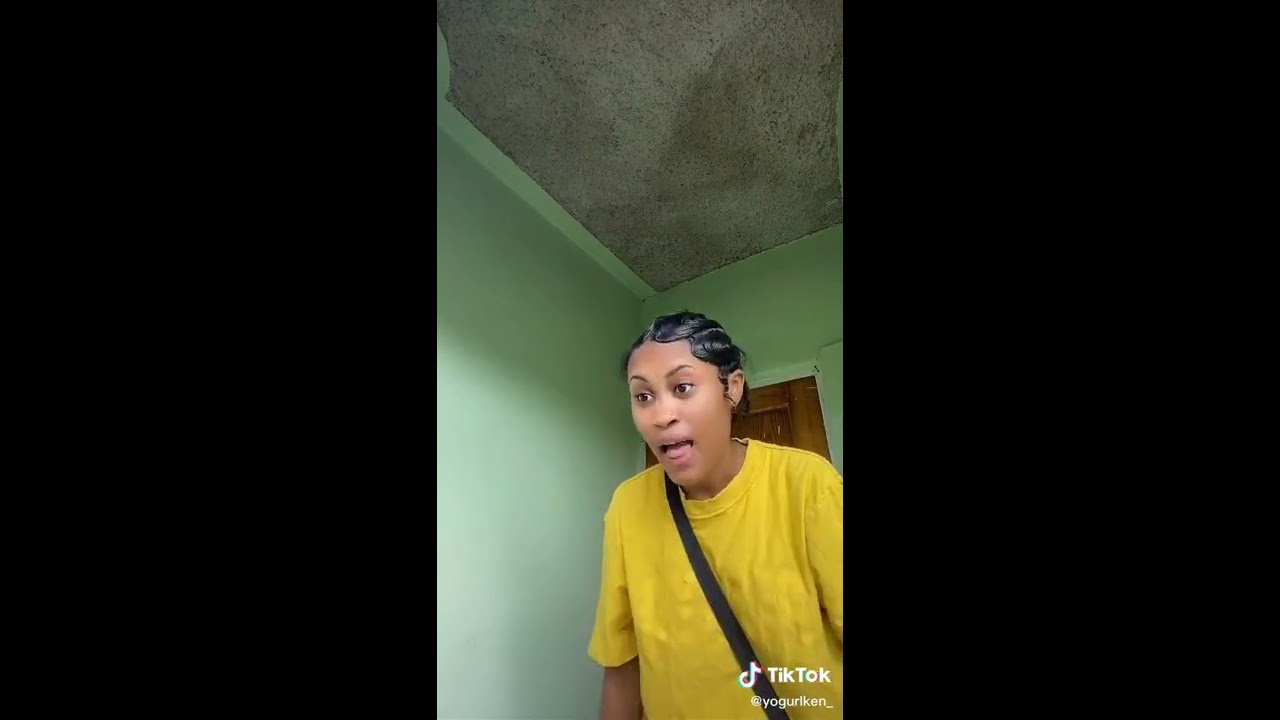The photograph features a young African American woman standing in a light green room with mottled gray ceiling. Dark wooden door frames, perhaps indicating a doorway, are visible behind her. She has short, wavy black hair styled reminiscent of Betty Boop. The woman is wearing a mustard yellow t-shirt with a strap over her right shoulder, her medium coffee-colored skin partially visible. Her mouth is slightly open as if speaking and her eyes wide with raised eyebrows, giving her an animated expression as though surprised or engaged. The right side of the image features a crack in the wall, and a TikTok logo is visible at the bottom right, suggesting the context might be social media. The image captures her from just above her breasts upwards, looking upwards at the camera.